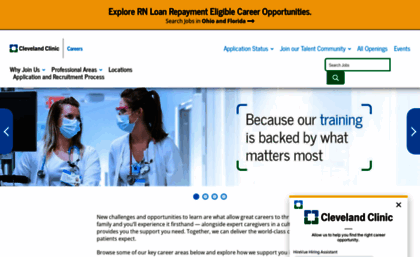The image is a screen capture of a web page with a clean white background that features various elements. At the top, there's a prominent yellow horizontal bar stretching across the entire width of the page, with black text that reads: "Explore RN Loan Repayment Eligible Career Opportunities." Directly below this bar, on the left side, there's a logo accompanied by some small, difficult-to-read text.

Central to the image are two women, both wearing blue face masks and white coats, suggesting they are healthcare professionals. The woman on the left has a blue and black stethoscope hanging around her neck. To the right of these women is a line of text that reads: "Because our training is backed by what matters most." The overall composition of the web page emphasizes a professional and supportive environment aimed at career advancement in nursing.